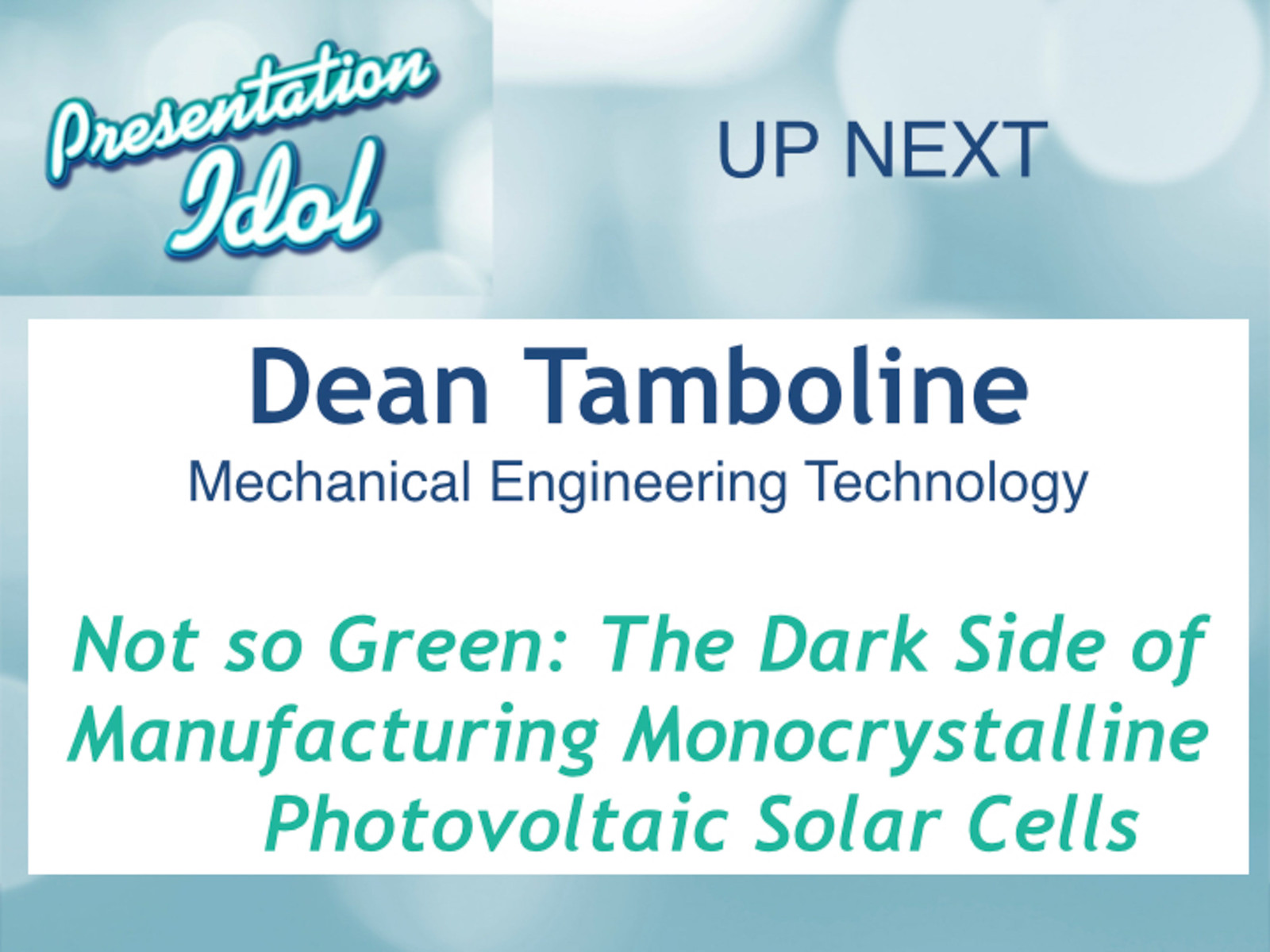The promotional banner features a light blue background adorned with various white bubbles, creating a soft, airy effect. Dominating the image is a large white rectangle that spans the bottom two-thirds, serving as the primary text area. 

At the top left corner of the image, amidst the blue background, the phrase “Presentation Idol” is elegantly written in white cursive text with a blue border. Just to the right of this, within the blue border, the words “Up Next” are displayed in a dark blue text. 

Prominently centered within the white rectangle, the name "Dean Tamboline" appears in bold blue font, along with the title "Mechanical Engineering Technology." Directly below, an italicized green text reads, “Not So Green: The Dark Side of Manufacturing Monocrystalline Photovoltaic Solar Cells.” This banner effectively combines various text colors and styles to convey detailed information about the upcoming presentation.